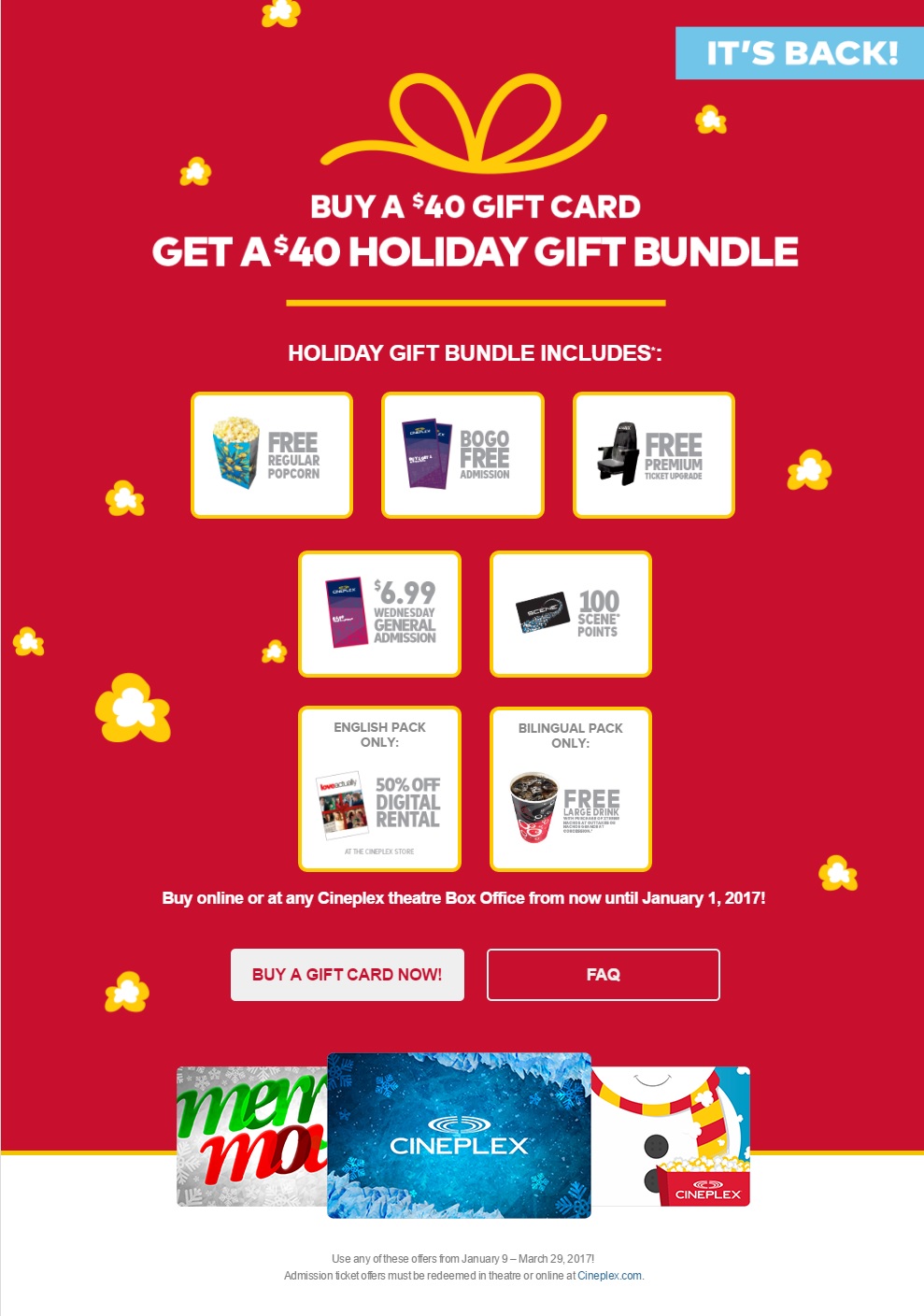Poster Description:

At the top right corner, the caption reads "It's Back!" in bold white text, drawing attention to the main promotion. The primary focus of the poster is a striking red background that features a large holiday-themed image. 

A vivid yellow ribbon starts from the left side and curves across the top of the poster. Along this ribbon, white text announces the promotion: "Buy a $40 Gift Card, Get a $40 Holiday Gift Bundle." 

The holiday gift bundle includes several exciting offers:
1. A bag of blue-packaged regular popcorn, outlined by a yellow border.
2. BOGO (Buy One, Get One) free admission tickets displayed prominently.
3. A free premium ticket upgrade clearly indicated within a yellow-bordered inset.
4. An offer for $6.99 general admission accompanied by an opportunity to earn 100 SCENE points.
5. An English pack-only card featuring nominal digital rental options and a bilingual pack-only card for large drinks.

Below these promotional items, further instructions are provided in white text: "Buy online or at any Cineplex theater box office from now until January 2017."

The central section of the poster proudly displays the Cineplex logo surrounded by a festive design featuring a green and red color scheme. To the right, an endearing snowman emphasizes the holiday theme.

At the bottom right, additional text notes that the promotion is valid from January 9 to March 29, 2017. It encourages customers to call for special duties or visit cineplex.com for more information.